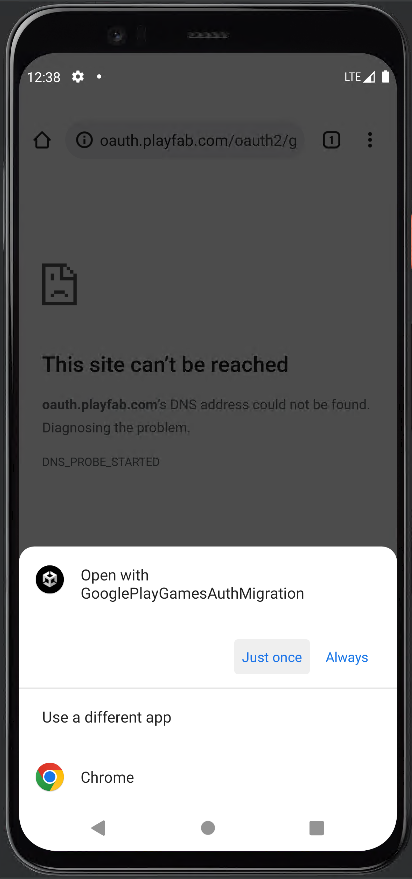This illustration features a close-up of a mobile phone with its screen prominently displayed against a dark grey background. The phone itself has a sleek black bezel, accented by a shiny grey line running along its edges. The top bezel is slightly thicker and houses a shiny grey lens positioned on the center left, accompanied by a horizontal row of grey dots in the middle.

The screen of the phone depicts a webpage with a darkened grey background. At the top left corner of the screen, there's a black home icon. To its right, a dark grey search bar contains black text reading "oauth.playfab.com/oauth2/g," though the complete URL is truncated on the right side of the bar. Adjacent to this, there's a black square outline with rounded corners featuring a black number '1' inside, followed by three vertically stacked black dots.

Below this, the webpage shows a pixelated icon on the top left, styled with a folded corner on the top right, and an eye with a frown on its face. Beneath the icon, bold black text reads "This site can’t be reached," followed by dark grey text detailing "oauth.playfab.com’s DNS address could not be found. Diagnosing the problem..." A smaller line of text directly underneath, "DNS_PROBE_STARTED," is separated by some negative space.

At the bottom of the screen, a white popup appears, containing unspecified text. This vividly detailed illustration captures the frustrating experience of encountering a DNS error on a mobile device, emphasizing the technical elements involved.